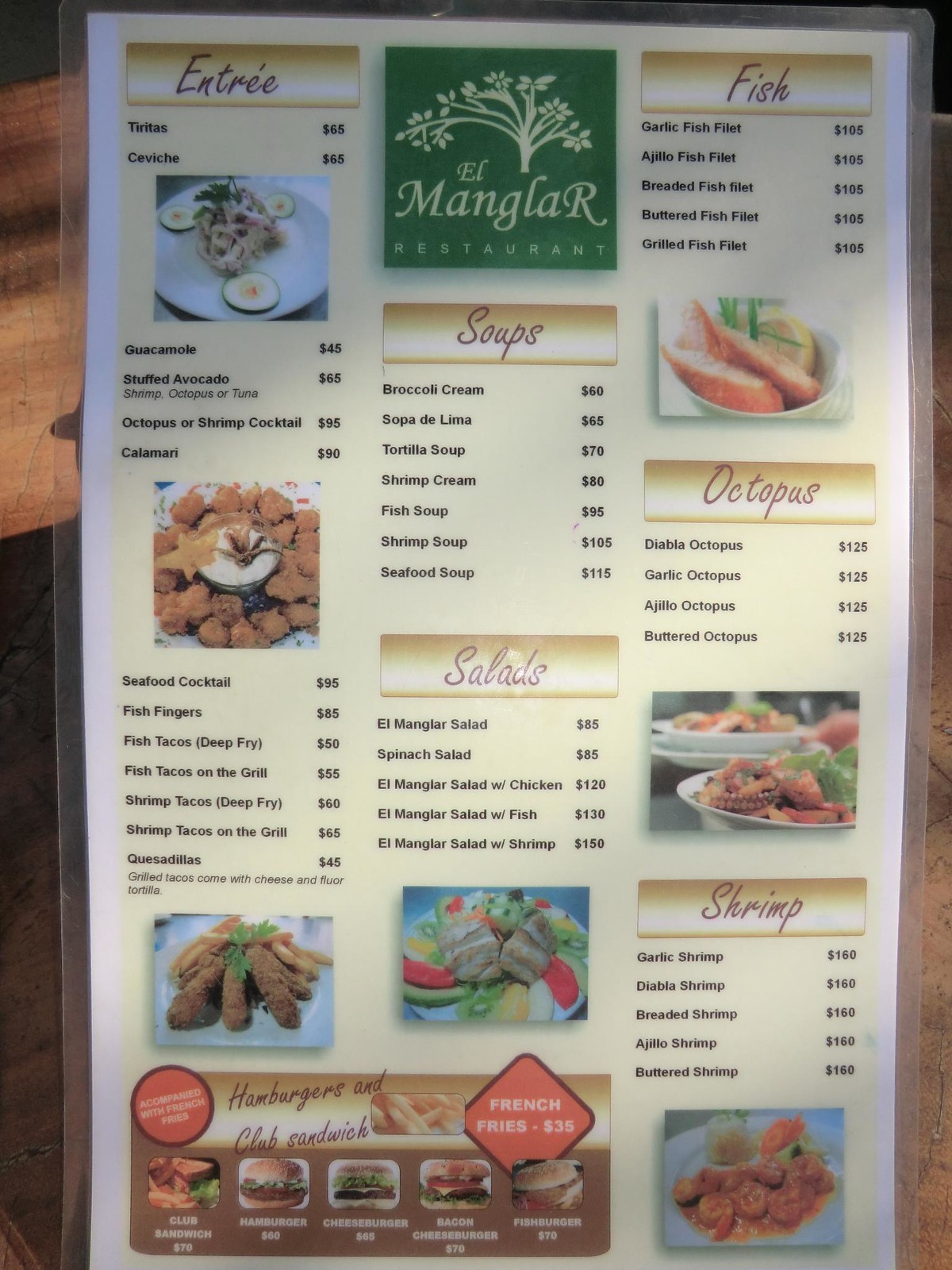This photograph captures the menu of El Manglar Restaurant, laminated with a thin, clear border framing its outer edges. At the top center of the menu is a green square featuring a cream-colored tree with a butterfly perched upon it, accompanied by the restaurant's name, "El Manglar Restaurant."

In the upper right-hand corner, the section titled "Fish" includes five entrée options. Directly below "Fish," the "Octopus" section offers four choices and features a picture of a dish showcasing calamari at its bottom. The "Fish" section has an image of salmon garnished with lemon.

At the bottom left, the "Shrimp" section lists five dishes, with a picture of shrimp served with an orange sauce displayed underneath. The central part of the menu highlights "Soups" with seven options and "Salads" with five. At the bottom of the "Salad" section, there's an image of a colorful fruit salad, featuring kiwi and various fruits.

The left side of the menu is dedicated to "Entrees," listing six choices along with a picture of a breaded dish. Additional options, around seven in total, are provided, with another image of a breaded item featured.

The bottom left-hand corner lists "Hamburgers and Club Sandwich" on a brown background, offering five variations and a side listing for French fries. The prices throughout the menu are not in U.S. dollars, as evident from items like French fries priced at $35 and a garlic fish filet costing $105.